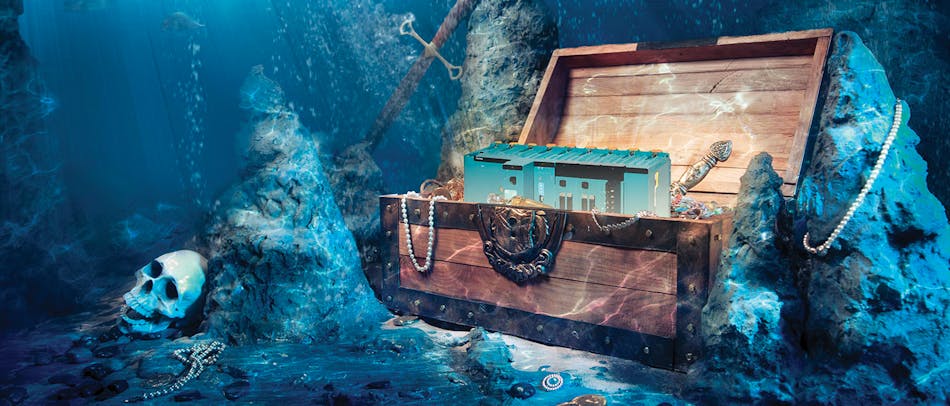The digital image depicts an underwater treasure scene at the ocean floor. Central to the image is an ornate wooden sea chest, partially open, revealing an array of treasures. The chest, which is accented with gold metal bracing and bolts, has another strand of pearls spilling out of it, along with some silver pieces. Inside the chest lies a mysterious blue, oblong object that does not appear to be aged or rusted. Leaning against the chest is the handle of a gold sword.

Surrounding the chest are various rock formations, with a prominent triangular rock to the left. Amidst these rocks rests a human skull, beside which a double-strand pearl necklace is delicately placed. Just behind the chest and slightly to the right, there is a rusted anchor encrusted with algae, though not fully visible. Another rusted sword is embedded in a stone nearby. On the right of the sea chest, a giant underwater stone features yet another pearl necklace elegantly wrapped around it, further emphasizing the abundance of treasure in this submerged scene.